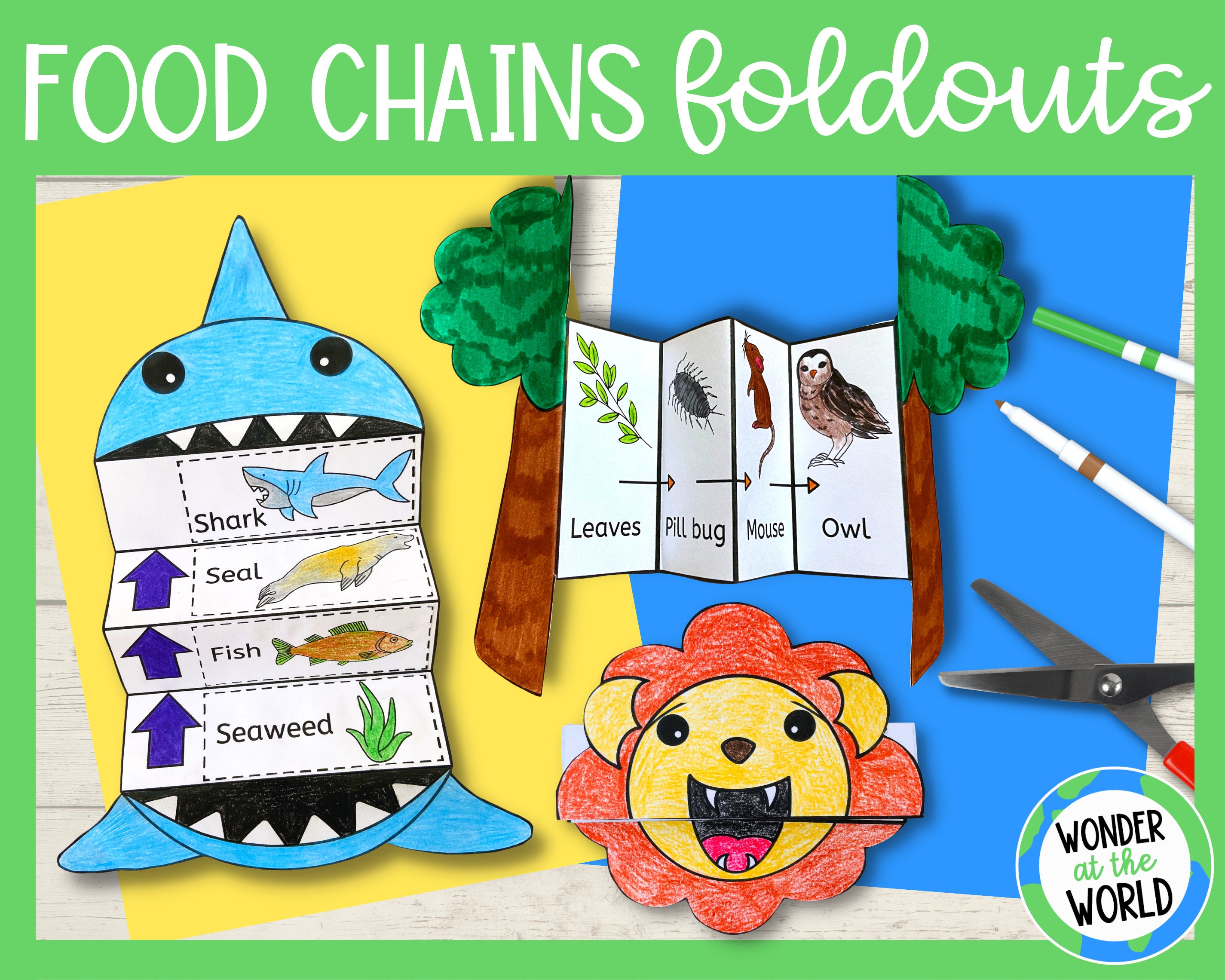The image is a colorful educational poster with a green trim border and a thicker green band at the top that reads "Food Chains Foldouts." Centered on the poster are various illustrated food chains designed for young learners. On the left, a cartoonish fish is shown with its mouth open, showing a multi-folded paper sequence: at the top is a blue shark, followed by an arrow pointing up to a yellow seal, then another arrow pointing up to an orange fish, and finally an arrow pointing up to green seaweed. In the middle of the poster, a tree illustration houses another fold-out paper, depicted with leaves at the top, followed by a sequence featuring a pill bug, a mouse, and an owl. Below this, there's a vibrant, cartoonish lion head with a yellow face and a red mane. To the right of these illustrations, the image includes a green marker, a brown marker with its cap off, a pair of rounded-edge scissors with red handles, and a small globe icon in the bottom right corner stamped with the words "Wonder at the World."